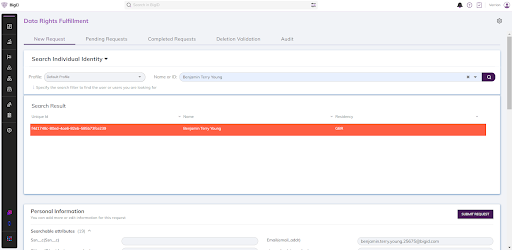The image depicts a detailed data management page. At the top, there is a section labeled "Data Flights for Humans." The bottom left corner features a segment for "Personal Information" and "Searchable Attributes." Towards the bottom right corner, an email address is shown, though the entry is either not visible or illegible. Additionally, the page includes a variety of search fields, complemented by subtext categories such as "New Requests," "Pending Requests," "Completed Requests," "Desktop Validation," and "Audits."